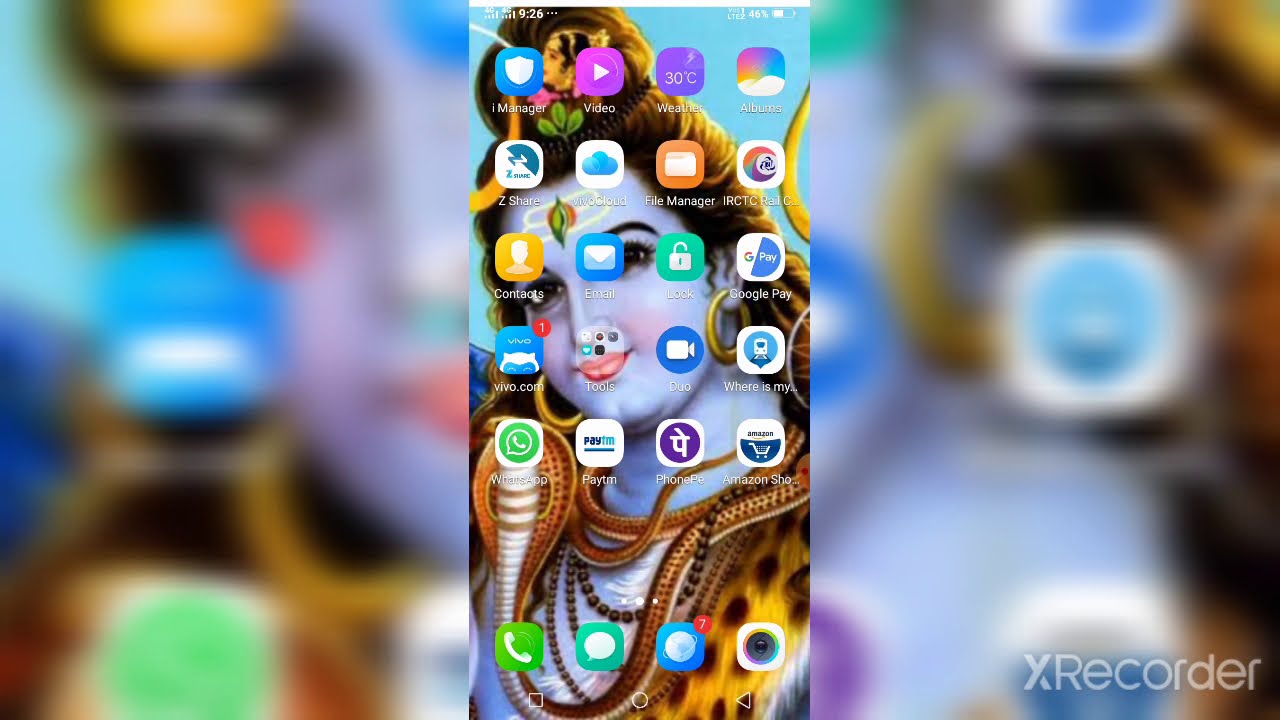This image appears to be a detailed screenshot of a smartphone's home screen, showcasing various apps and a vivid, spiritual-themed background. The wallpaper features an Eastern spiritual deity or goddess with striking purple skin and an ornate appearance. She is adorned with gold earrings, a cheetah-patterned vest, snakes draped around her neck, and flowing golden hair. Her lips are painted pink and her presence embodies a mystical aura.

The home screen is organized with apps arranged in a grid formation, specifically five rows by four columns, with an additional row at the bottom dedicated to essential apps like phone, messages, web browser, and camera. Among the diverse apps present are iManager with a blue shield, VideoApp with a purple play button, Weather displaying 30 degrees, Albums, Zshare, iCloud, File Manager, IRTC, Contacts, Email, a green lock app, Google Pay, Vivo, Tools folder, Duo with a camera icon, WhatsApp, Paytm, Amazon Shop, and several more.

At the top of the screen, the time reads 9:26, and the battery life is indicated at 46%. The overall scene is set against the dynamic background of the purple-skinned goddess, who adds a sense of depth and allure to the smartphone’s display, intertwined with the colorful apps that range from blues and purples to yellows, greens, and whites. The image is further anchored by some on-screen text in the lower right corner, which reads "X recorder," hinting at a screen recording in progress.